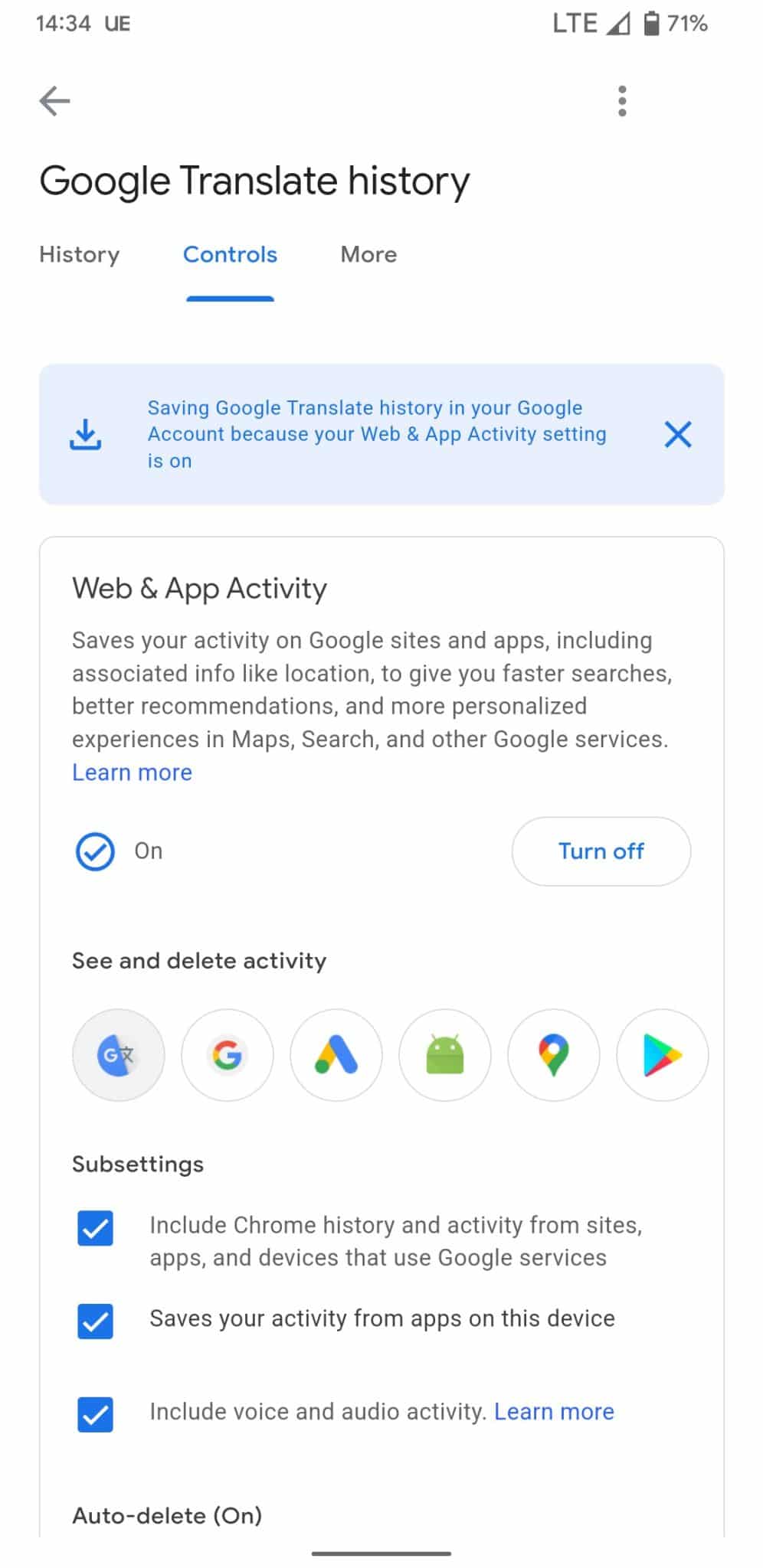The image displays a Google settings page with a white background. At the top, the status bar shows "1434 UE" on the left, and on the right, there is an LTE indicator with a partially filled data icon and a battery icon showing 71% charge. 

Below the status bar, the header reads "Google Translate History" with three options: Histories, Controls, and More. The "Controls" option is highlighted in blue and underlined to indicate it is selected. 

The page explains that Google Translate history is being saved to your Google account because the "Web & App Activity" setting is enabled. It highlights that when this setting is on, your activity on Google sites and apps, along with associated information like location, is saved to provide faster searches, better recommendations, and more personalized experiences across Google services such as Maps and Search. There is a "Learn more" link in blue text for further information. 

The option to turn off this setting is indicated by a white button with blue text labeled "Turn Off". 

Additionally, the page offers options to see and delete activity, represented by various icons including the Google logo, an upward-pointing arrow, the Google Maps icon, the Play Store icon, and the Android icon. 

Under "Sub Settings," the following options are outlined with blue checkmarks next to them:
- Include Chrome history and activity from sites, apps, and devices that use Google services.
- Save your activity from apps on this device.
- Include voice and audio activity.

Finally, "Auto-delete on" is mentioned at the bottom of the page.